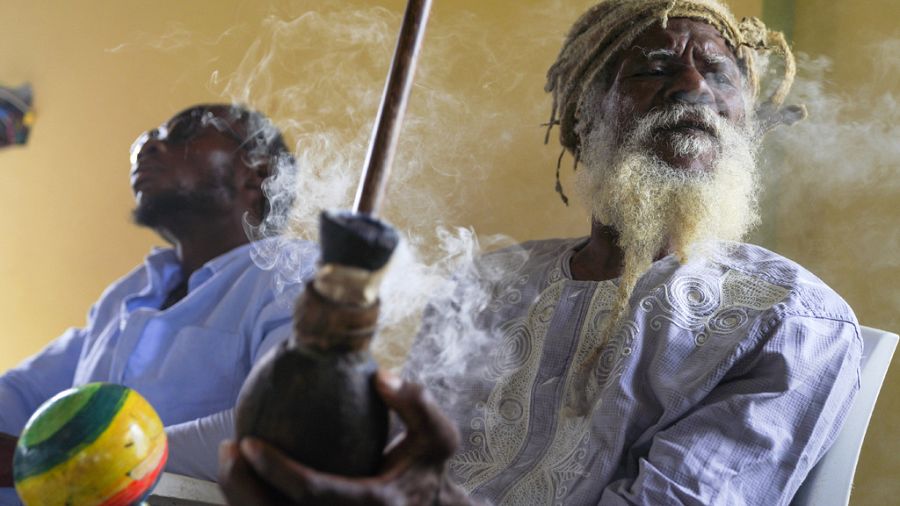This photograph captures a poignant moment between two African men, possibly engaged in a ceremonial act, as they smoke from a large black pipe. In the foreground, an elderly man exudes wisdom with his white beard, dreadlocks peeking from under a straw hat, and traditional African attire—a light blue shirt embellished with white swirly embroidery. He's deeply focused, exhaling a plume of smoke which envelops his weathered face. At his side, seated slightly further back, is a younger man adorned in a modern light blue button-down shirt with a collar. He sports a lighter beard, wears glasses, and leans back in a relaxed pose, savoring the moment with a contemplative gaze. Both are seated on white chairs against a backdrop of yellow walls, illuminated by sunlight streaming in from both sides, casting a serene glow over the scene.